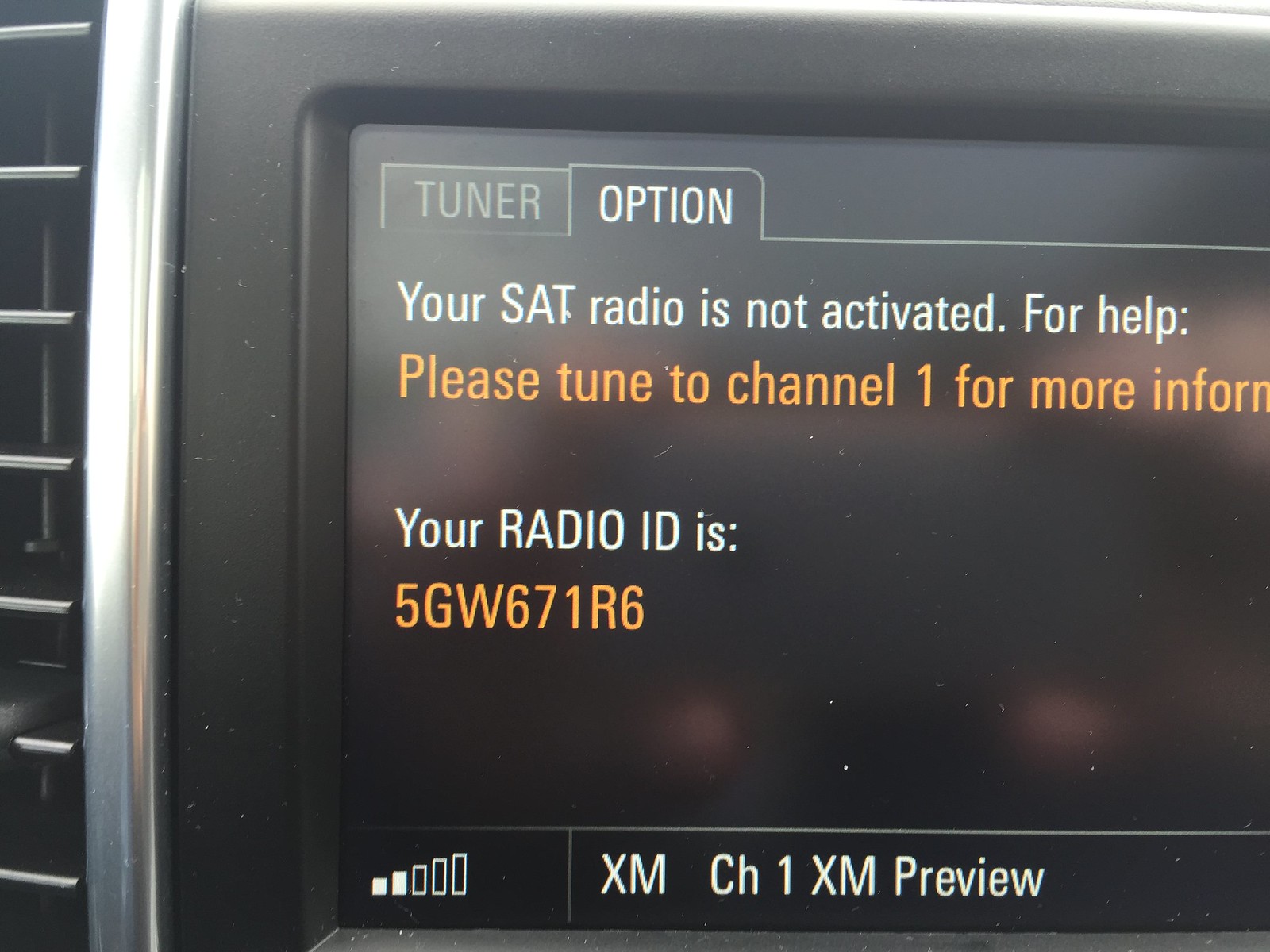Caption for the Image: 

"The interior of a car displaying the XM Satellite Radio system on the dashboard screen. The message on the screen reads, 'Your satellite radio is not activated. For more help, please tune to channel 1 for more information.' Below this message, the radio ID is visible: 5GW671R6. The interface also indicates a channel preview option, suggesting that once the satellite radio is activated, users will be able to switch between channels. The setup is ready to offer an array of satellite radio channels, provided that activation steps are followed by tuning into channel 1."